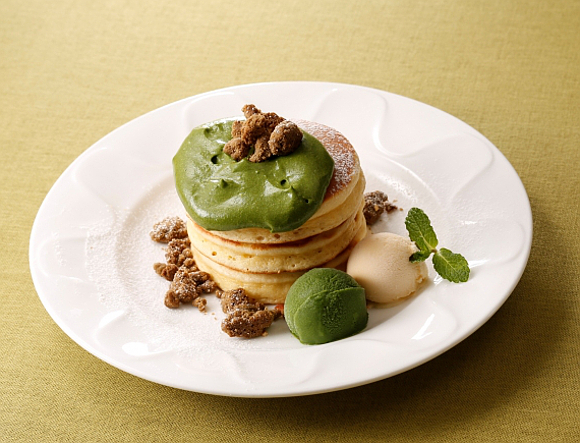The image depicts a meticulously arranged plate of food set on a cream-colored napkin or table. The plate itself is white with a looping design on its outer rim, which remains mostly uncovered but for a small green leaf garnish. The focal point of the dish is a trio of small, coin-sized pancakes positioned in the center of the plate. These pancakes are topped with a dusting of powdered sugar and a green sauce, which could be a gooey garnish or perhaps avocado. Sprinkled around the pancakes are what appear to be caramelized pecans or crushed nuts, adding a brown, crumbly texture to the presentation. Beside the pancakes is a small pile of a green mixture, which resembles ice cream or a green sauce, and a perfectly round, white scoop that looks like butter with a green leaf sticking out of it. This juxtaposition of textures and colors suggests a dessert-like dish with a unique, savory twist.